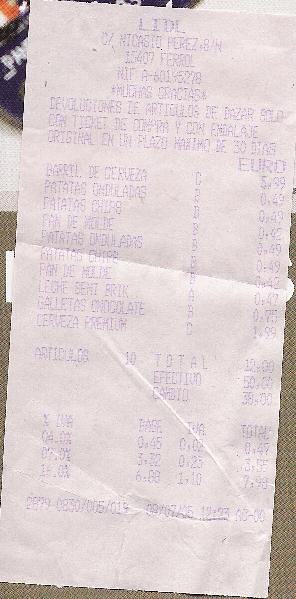This image features a photograph of a highly faded receipt, likely from a grocery store or similar establishment. The receipt itself is on white paper with blue ink, though the text and numbers have become so faint over time that they are nearly unreadable. At the top of the receipt, the possible store name "LIDL" is somewhat discernible, suggesting it may be from a location bearing that name. The overall condition of the receipt, with its considerable fading, obscures any further specific details about its contents.